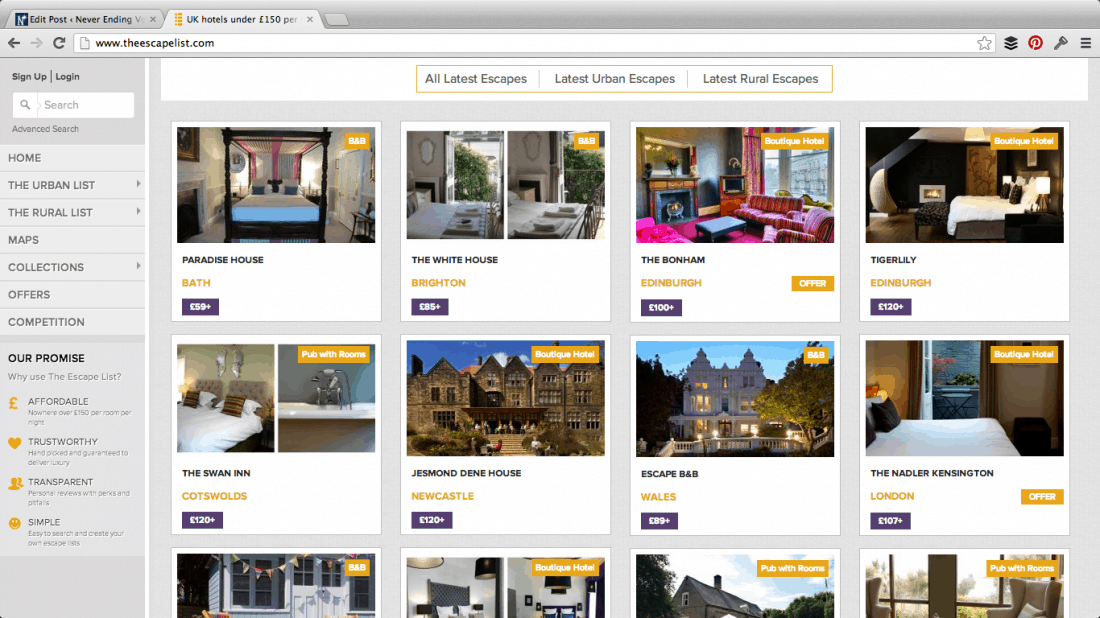This is a detailed screenshot of a travel website specializing in vacation escapes. The active browser tab is titled "UK Hotels Under £150 per Night." Below the tab is the website address bar displaying "www.theescapelist.com." To the left of the address bar, there are refresh and back buttons, while to the right are icons for various applications, including Pinterest and utilities.

On the left side of the screen, a gray vertical navigation bar is visible. At its top, there are "Sign Up" and "Log In" options, followed by a white search bar. The main navigation categories listed in uppercase black font include "HOME," "THE URBAN LIST," "THE RURAL LIST," "MAPS," "COLLECTIONS," and "OFFERS AND COMPETITIONS." Further down are sections labeled "OUR PROMISE," "WHY USE," and "THE ESCAPE LIST," each accompanied by mustard gold icons. Four reasons are listed: 
1. A pound sign for "Affordable,"
2. A heart for "Trustworthy,"
3. Two profile heads for "Transparent,"
4. A circle for "Simple."

In the main content area, twelve images of destinations are displayed, eight fully visible and four partially. These images showcase various destinations, indicating their names such as "Paradise House," locations (e.g., Bath, Brighton, Edinburgh, Cotswolds, Newcastle, Wales, London), and nightly costs within blue (navy blue) bars. Some of the images feature banners in the top right corner with special notices like "Offer." The images are a mix of exterior shots and interior shots of the accommodations.